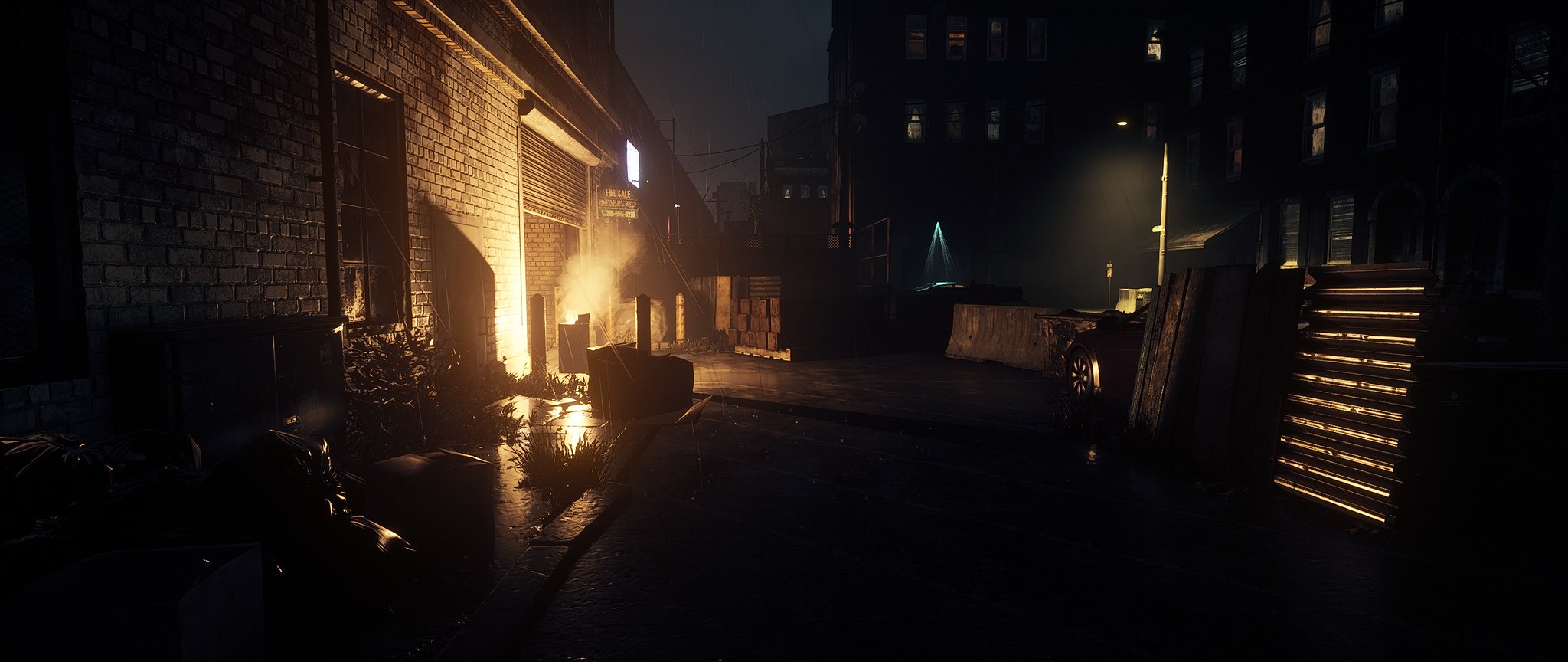This photograph, taken at night, captures a moody industrial alleyway scene. On the left side of the image, a brick building stands in partial darkness, illuminated by a soft amber-white light casting a warm glow on its facade. On the ground beside the building are several black trash bags, adding to the gritty ambiance. Some resilient bushes peek through cracks in the concrete, adding a touch of nature amidst the urban setting. In the background, tendrils of smoke suggest that something is on fire, adding a layer of tension and mystique to the scene. 

To the right, a section of corrugated metal is visible, along with a partial view of a parked car, which hints at the area's functionality. A single street lamp casts its light, contributing to the interplay of shadows and illumination. Further along, additional buildings are visible, their windows glowing with a soft, pale orange light that contrasts with the night's darkness. Overhead, power lines crisscross the sky, while a concrete barrier delineates space within the alleyway. The composition of elements—the light, smoke, and urban textures—creates a vivid and detailed nighttime tableau.